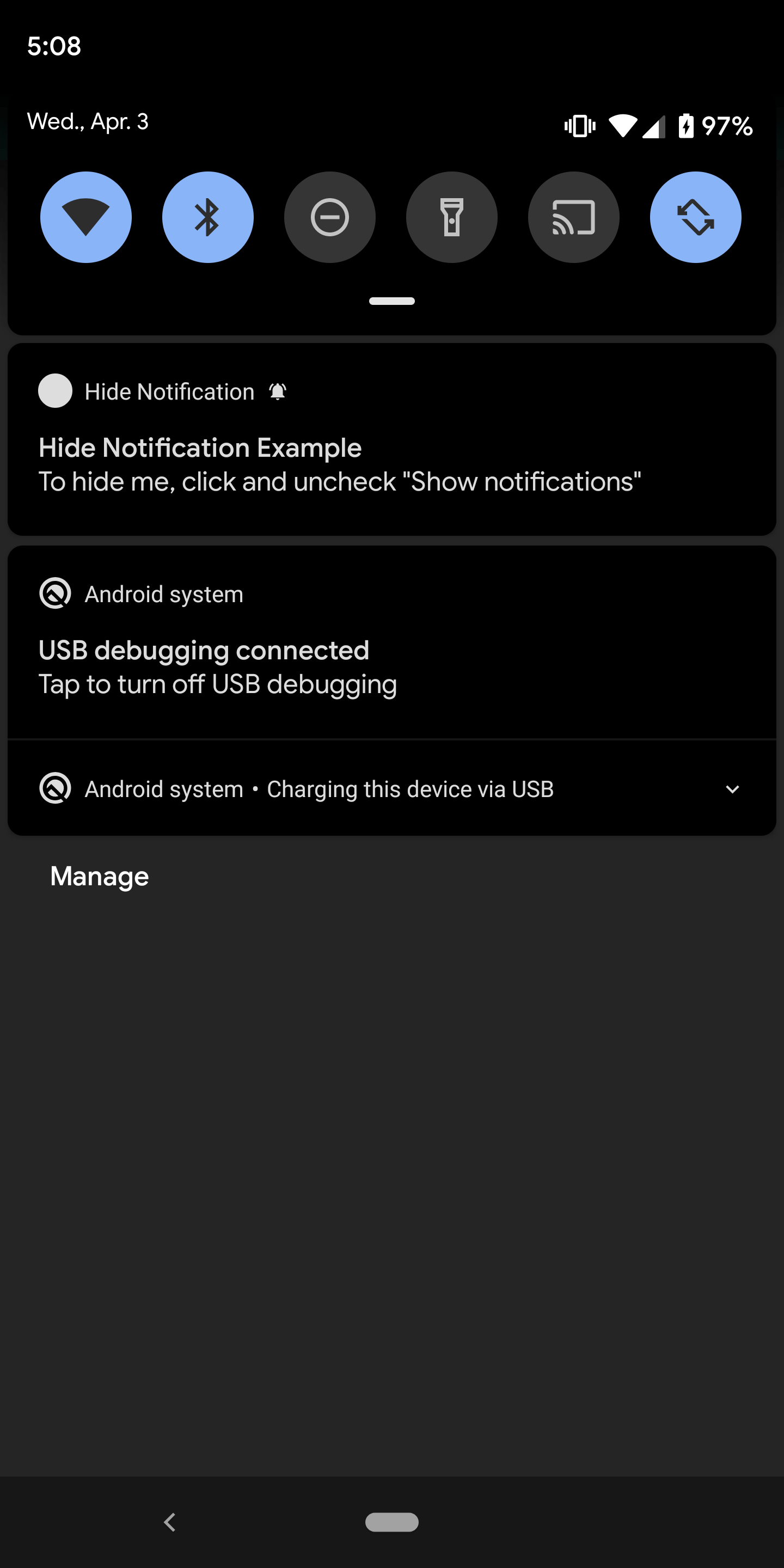This detailed screenshot captures the interface of an Android cell phone application in dark mode. The background is entirely black with gray tones, and the text is displayed in white for high contrast. The screenshot prominently displays a minimalist design, devoid of specific images, focusing solely on standard cell phone icons and notifications.

In the top left-hand corner, the time is indicated as 5:08, although it is unclear whether it is AM or PM. Directly below the time, the date is stated as Wednesday, April 3rd, albeit without specifying the year. The status bar at the top shows several system indicators: the phone is in vibrate mode, the cell signal strength is visible, the Wi-Fi is connected, and the battery is currently at 97%.

There are six distinct icons representing various settings and features. Three of these icons are currently active: Wi-Fi, Bluetooth, and a third icon featuring two arrows, which might indicate synchronization or data usage. The remaining icons are for streaming, the flashlight, and possibly other utilities. The presence of quick toggles for starting and stopping applications suggests an emphasis on user convenience and efficiency, which is characteristic of Android devices.